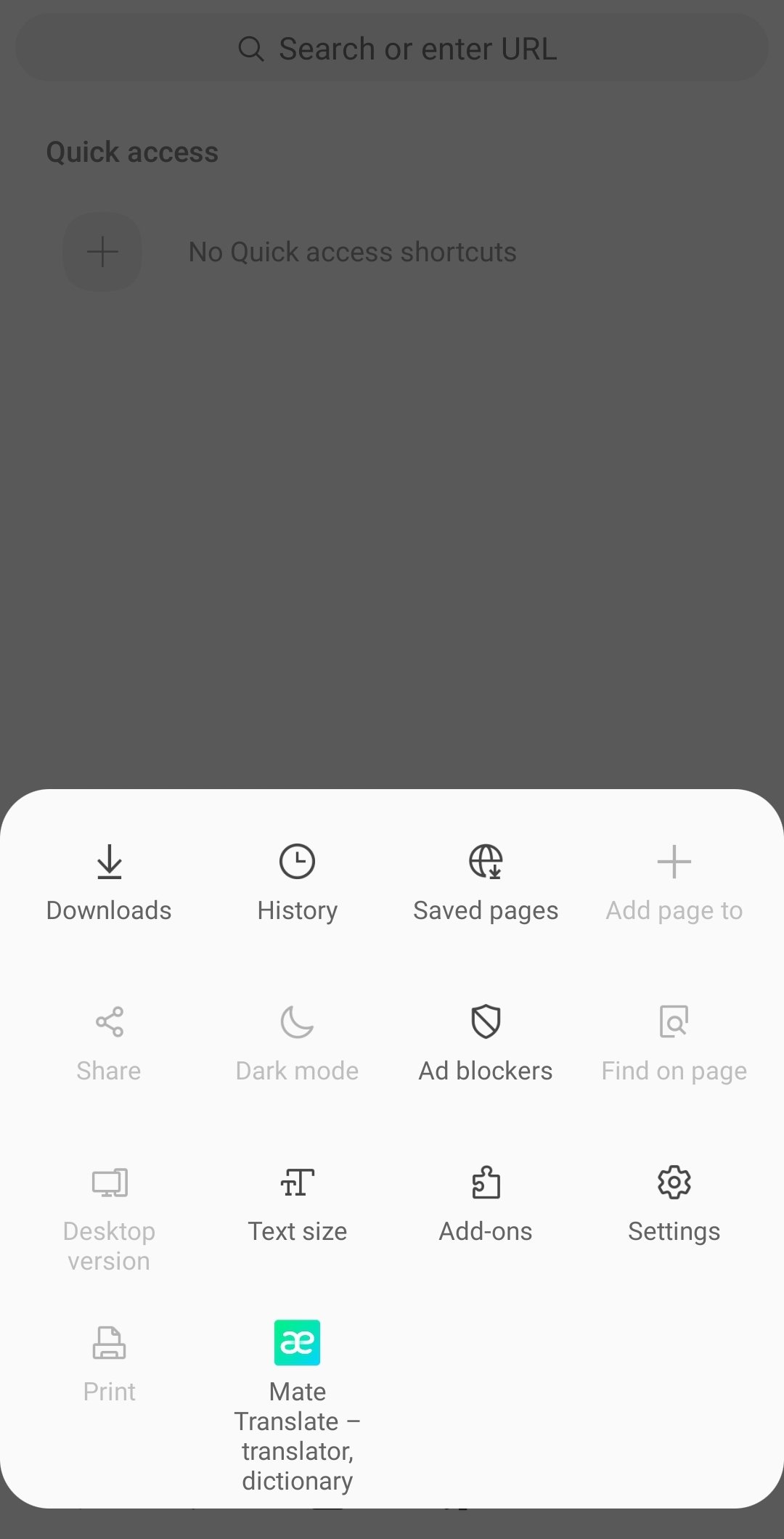In this detailed image, the top section features a blurred gray background with various UI elements, including a central text that reads "Search for inner URL". Directly beneath this, the words "Quick Access" are visible, followed by a plus button icon. However, these elements are not the primary focus of the image.

The central and most prominent part of the image is located at the bottom, highlighted with a white background and black text. This section is organized into several rows with distinct functionalities. Starting from the left, the first row includes options like "Downloads", "History", and "Saved Pages", each labeled clearly. To the right of these options is a plus icon labeled "Add Page".

The second row features important tools such as "Share", a button marked "Dark Mode" with a moon icon, an "Ad Blocker" indicated by its symbol, and "Find on Page" marked with a search icon.

Following this, the third row lists further options: "Desktop Version", "Text Size", "Add-ons", and "Settings", each accompanied by their corresponding icons.

In the subsequent row, there is a "Print" option, and next to it, the "Mate Translate - Translator Dictionary" option, which is denoted by two distinct icons supporting the functions of translation and dictionary lookup.

Overall, the image compartmentalizes various useful browser and device functionalities into a clear, structured layout at the bottom, making these tools readily accessible to the user.